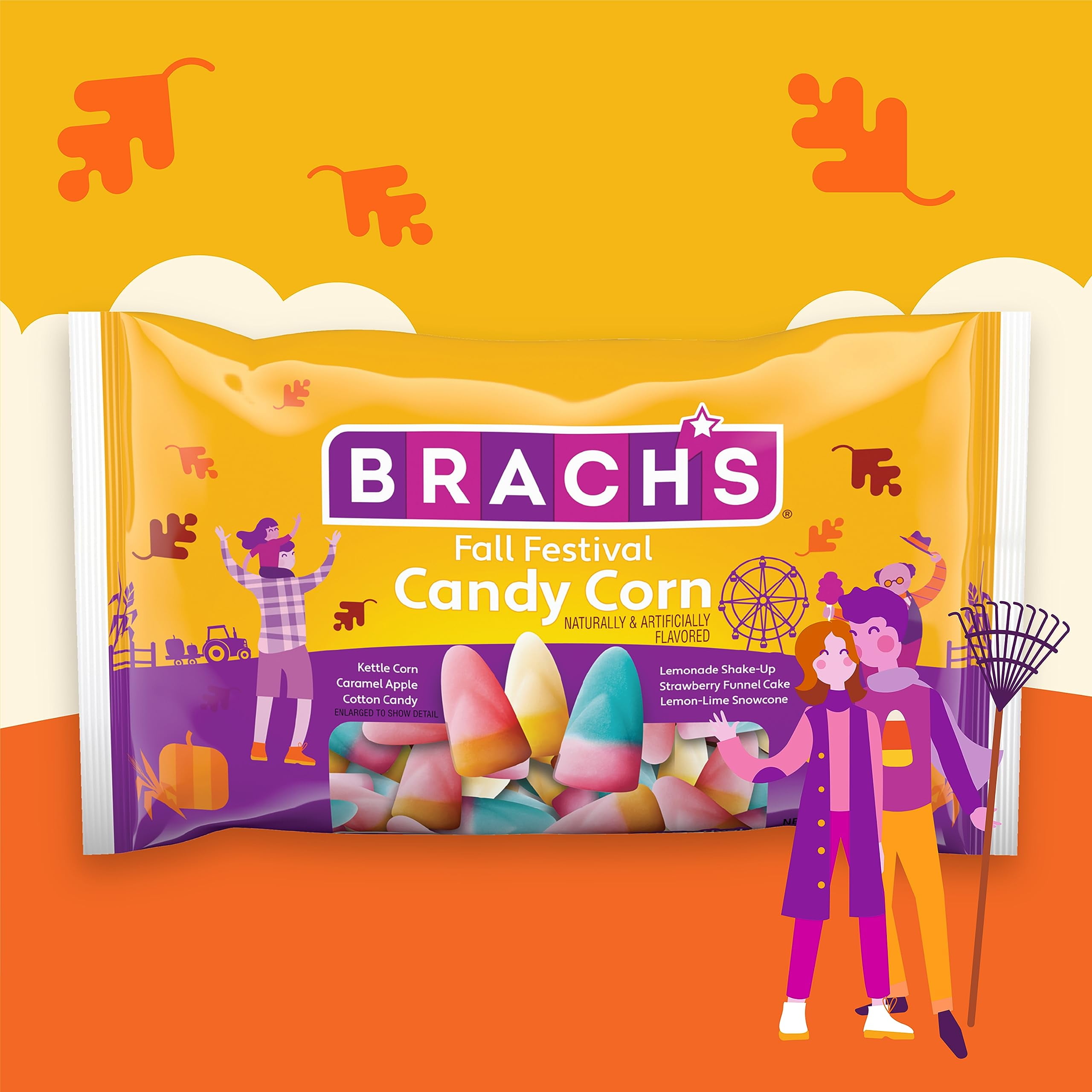The image prominently displays a bag of Brock's Fall Festival Candy Corn, featuring a variety of flavors such as kettle corn, caramel apple, cotton candy, lemonade shake-up, strawberry funnel cake, and lemon-lime snow cone. The candy corn comes in an array of colors from yellow and purple to pink, orange, blue, and white. The bag, labeled "Brock's" in white lettering with a star for the apostrophe, is adorned with autumnal elements like orange and brown leaves that appear to float. The background transitions from gold with leaf patterns at the top to orange at the bottom. Surrounding the bag are animated festival scenes: a dad with a child on his shoulders, a tractor, a fence, a ferris wheel, and a bald man raising his hat. Additionally, a cartoon couple is featured, with the man in yellow pants and a patterned purple sweater kissing a woman in fuchsia pants and a purple vest, capturing the essence of a festive fall celebration.